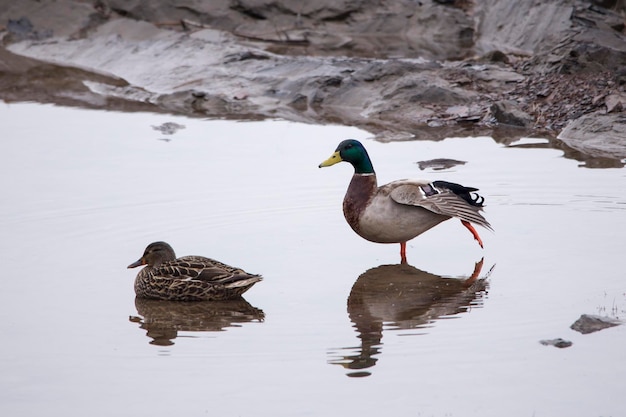In this rectangular photograph, we see two mallard ducks—a female on the left and a male on the right—amidst a serene water body that appears brown due to the low depth. The female mallard, with brown and white plumage accented by tan, khaki stripes, is sitting down in the water, casting a clear reflection. The male mallard, characterized by his striking green neck, yellow beak, brown chest, white wing tips, grayish body, black tail, and distinctive orange legs, stands on one leg in the shallow water, with his left leg lifted suggestively as if he's stretching or preparing to walk. The background features an assortment of gray rocks, some smooth and some sharp, that meet the edge of the water, underlying the natural setting of this tranquil scene. The overall gray tone of the image suggests overcast skies, possibly hinting at a winter day.